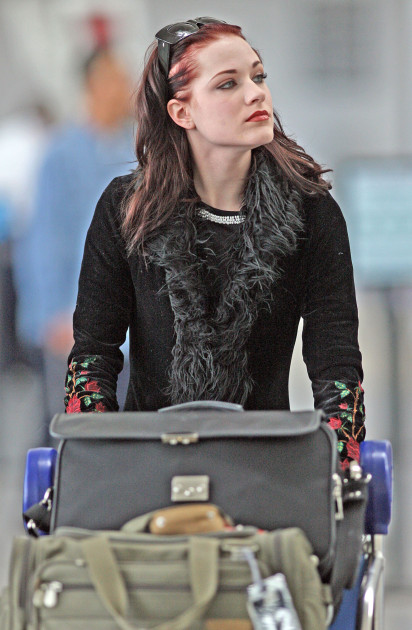The photograph features a young Caucasian woman in her late 20s or early 30s, who is likely at an airport, pushing a medium blue luggage cart. The cart has two large bags on it, one gray and the other olive green. The woman, with a pale complexion, has long, reddish-brown hair that appears to be dyed to accentuate the red tones. She is wearing black sunglasses perched on top of her head, along with eyeshadow and lipstick. Her attire includes a long black top with a furry neckline and ornate sleeves adorned with red and green floral designs, possibly roses or ivy. Completing her outfit is a light black jacket that also features floral patterns on the lower sleeves and fur or faux fur along the collar and chest. The background is blurred, focusing attention on her and the luggage cart.